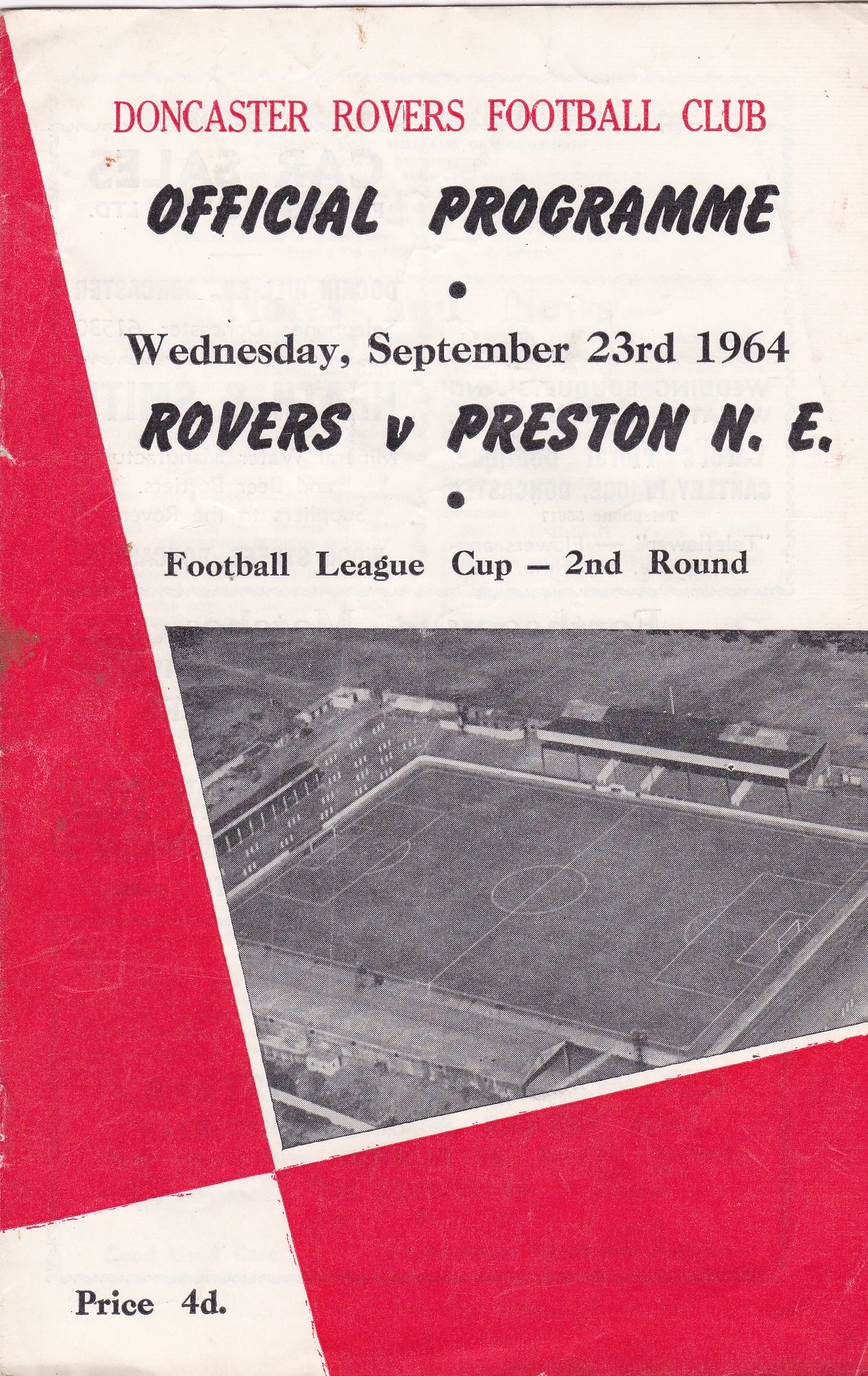This image features the aged and yellowed front cover of an official program for a soccer match, specifically for the Doncaster Rovers Football Club. The background predominantly displays white with red geometric shapes, including a triangle along the left edge joining a section along the bottom right. Across the top, bold red text proclaims "Doncaster Rovers Football Club," followed by "Official Program" in black text. Further details state the event occurred on "Wednesday, September 23, 1964," and involved the "Rovers v. Preston N.E." in the "Football League Cup, 2nd Round." Centrally positioned is a black-and-white photograph of an empty football pitch taken from an aerial perspective. In the bottom right corner of the cover, the price is indicated as "Price 4D" in black text. The entire layout and graphic elements suggest a classic, historical design typical of mid-20th-century sports memorabilia.